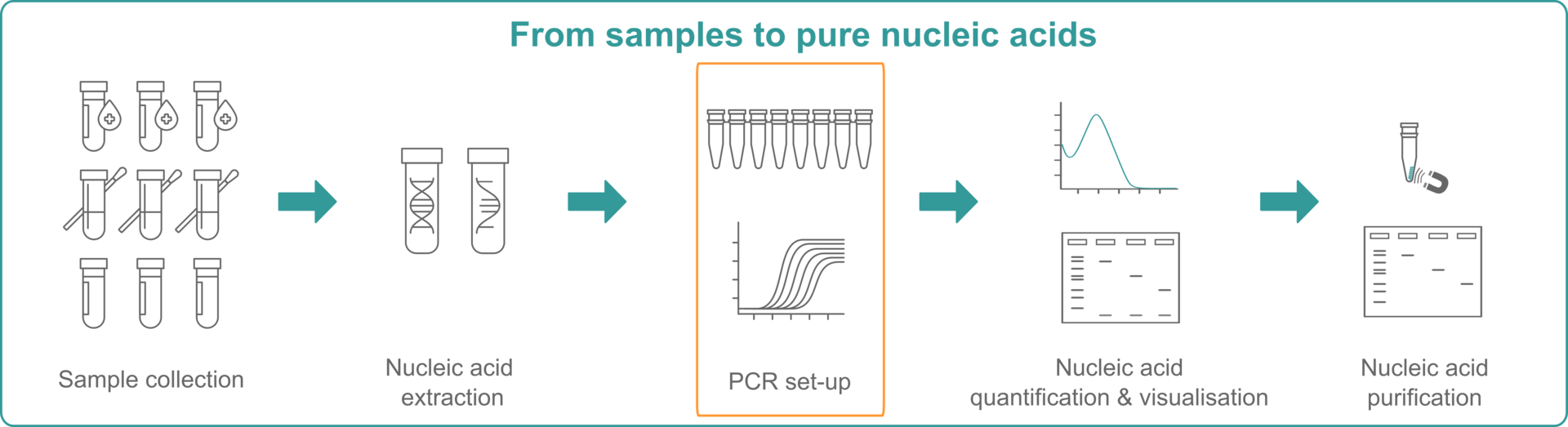This detailed black-and-white diagram, accentuated with green arrows and a green title, illustrates the process titled "From Samples to Pure Nucleic Acids." The first step, "Sample Collection," features nine dark gray, animated test tubes. Progressing to the second step, "Nucleic Acid Extraction," fewer test tubes are depicted, accompanied by a DNA symbol. The third step, highlighted within an orange box, is "PCR Setup," showing various scientific objects with curving lines and graph elements. The fourth step, "Nucleic Acid Quantification and Visualization," includes a square with dots and a singular blue line going down a graph. The final step, "Nucleic Acid Purification," features a scientific tube, a square diagram, and is marked by a blue outline. Each step is connected by rightward-pointing blue arrows, clearly defining the workflow from the initial sample collection to the final purification of nucleic acids.